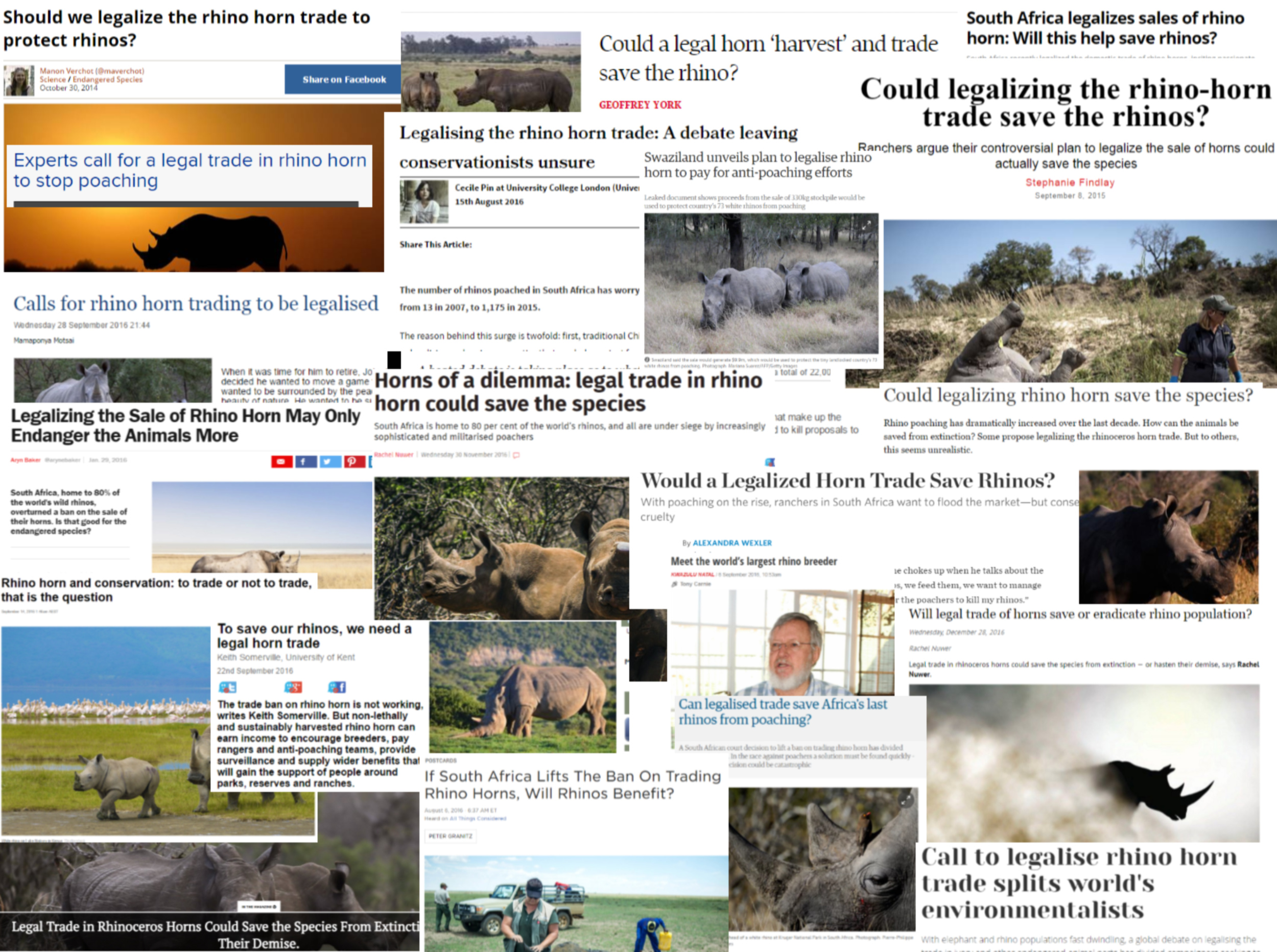The screenshot captures a webpage from a computer, densely packed with images and headlines focusing on the controversial topic of the rhino horn trade. In the top left, a headline reads, "Should we legalize the rhino horn trade to protect rhinos?" To its right is a photograph of a rhino in its natural habitat. The upper right corner features a headline stating, "South Africa legalizes sales of rhino horn. Will this help save rhinos?" Alongside this text is another rhino image, this time at sunset, framing the creature against a striking orange sky with the caption, "Experts call for a legal trade in rhino horn to stop poaching."

Additional images and headlines are scattered throughout the page. In the middle right, middle, and bottom sections, more pictures of rhinos appear. The bottom left displays a rhino enveloped in a cloud of smoke, underscored by the words, "Call to legalize rhino horn trade splits world's environmentalists." Directly above it, another tagline poses the question, "Will legal trade of horns save or eradicate rhino population?" Together, these elements create a mosaic that visually and textually debates the implications of legalizing the rhino horn trade.